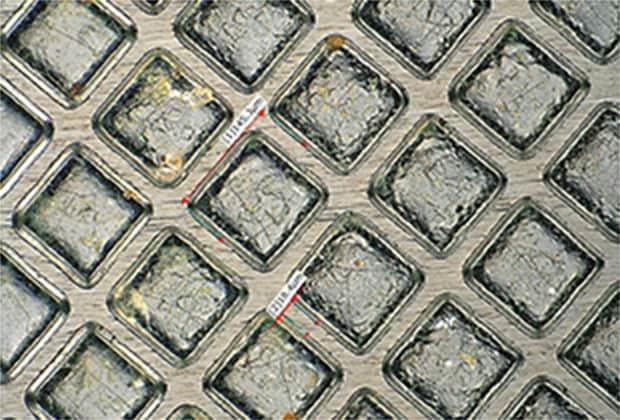The image depicts a highly zoomed-in view of a diagonal grid pattern in light gray tones, possibly made of concrete, stone, or metal. The grid features a lattice design with small recessed squares between the lines, giving it a textured, stone-like quality. Among the grid's diagonal lines, some of which appear metallic or ice-like, there are digitally-added red and blue lines; the red lines stretch diagonally, while the blue lines, each with red dots at the ends, run perpendicularly to them. Two small, blurry sticker labels, which could have faint black text, are affixed near the center. The image includes subtle accents of gold and pale green that add to its abstract, artistic nature. The horizontal grain visible in the lattice gaps between the diamonds enhances its complex, detailed appearance.